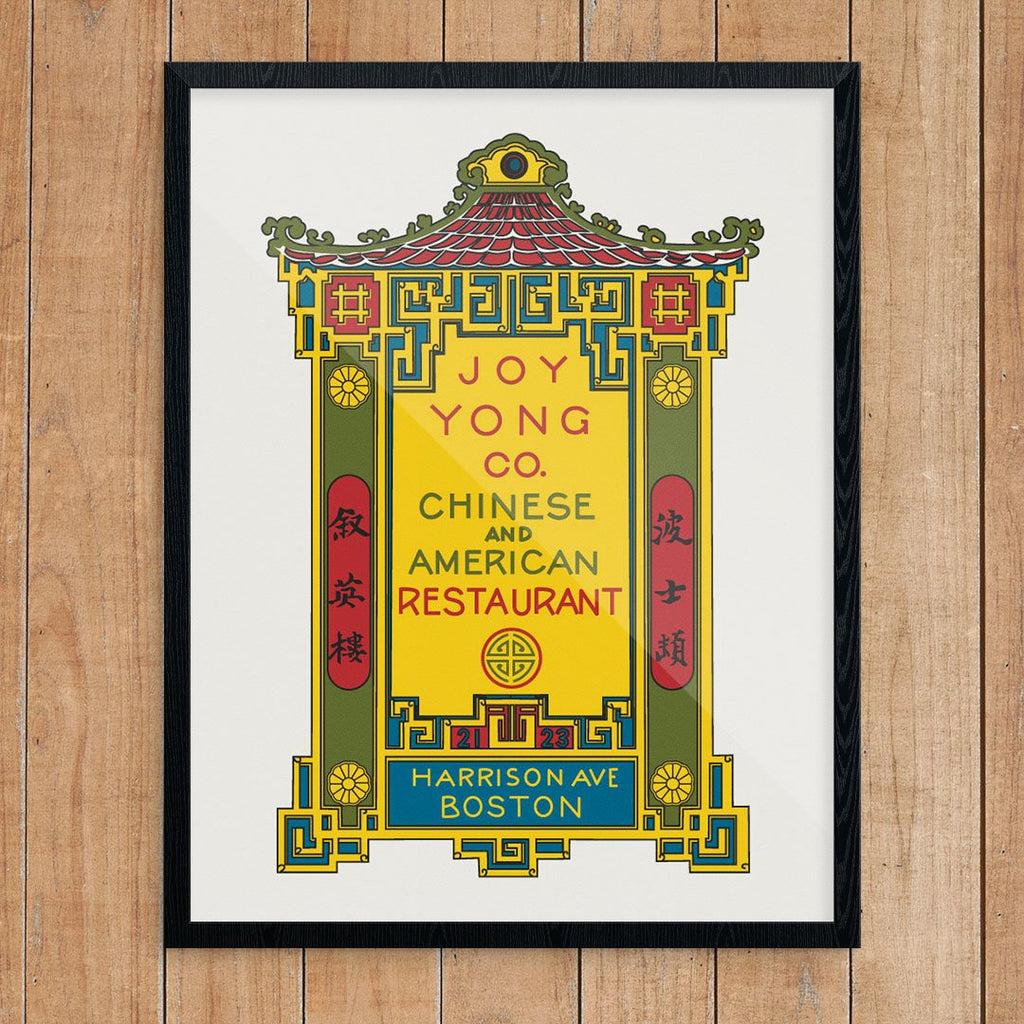The photograph showcases a framed illustration laid against a background that resembles wooden flooring or paneling. The vibrant artwork prominently features the name "Joy Yong Ko, Chinese and American Restaurant," suggesting it is likely one of the pioneering Chinese restaurants on Harrison Avenue in Boston. The illustration exudes a traditional Chinese aesthetic, possibly inspired by a Chinese building or temple, and is rich with vivid colors such as yellow, green, blue, and red. Flanking the central text are Chinese characters, one on either side, that add to the authentic cultural ambiance of the piece. This meticulously composed image captures the essence of early Chinese-American culinary heritage with its blend of ornate design and historical significance.